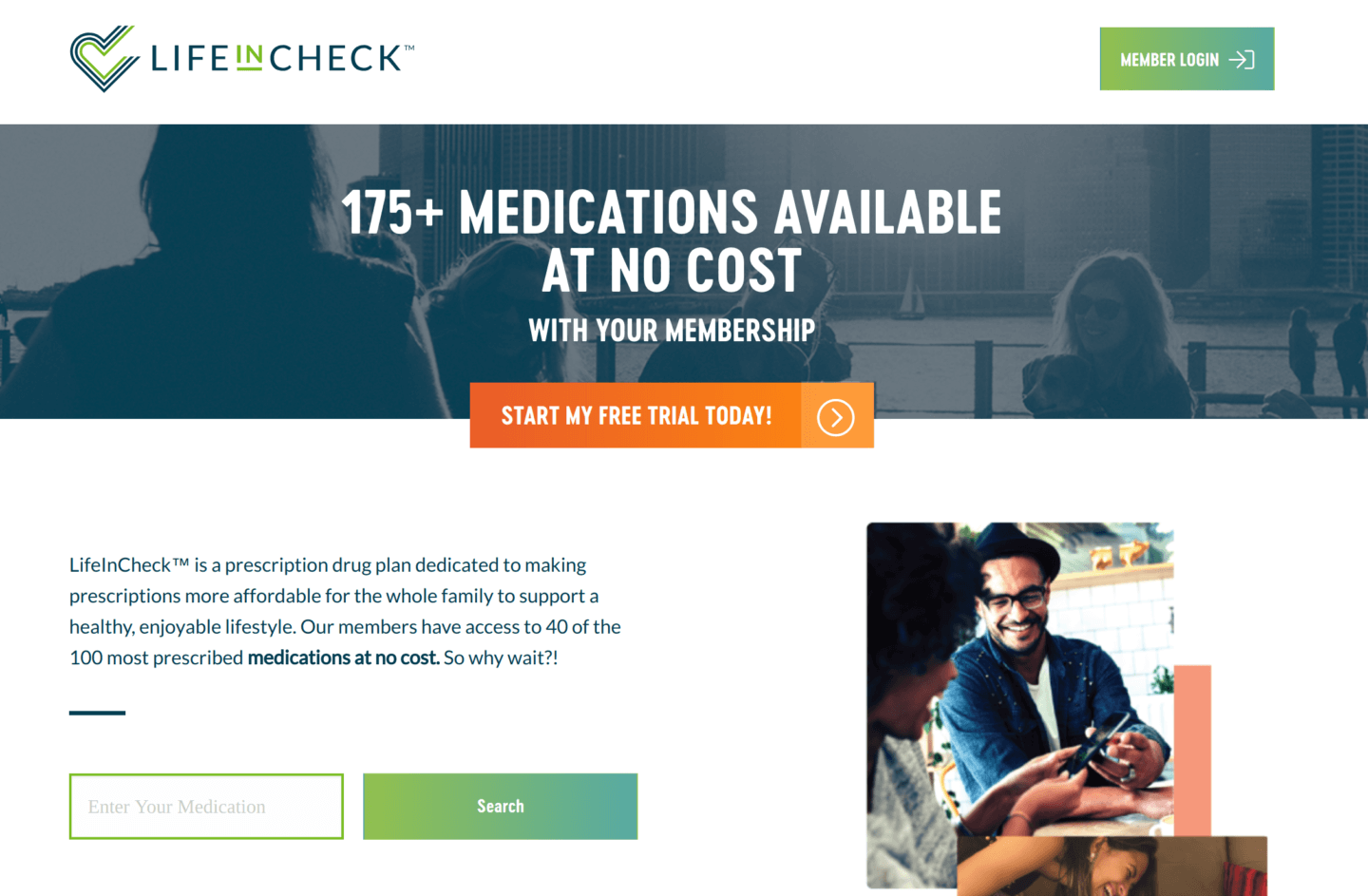The image showcases the Life in Check prescription plan, aimed at making medications more affordable for families. 

In the top left corner, the Life in Check logo and name are prominently displayed. Opposite, in the top right corner, a green rectangle labeled "Member Login" is visible. Dominating the center of the page is a dark, shadowy photograph featuring several individuals. On the far right, a woman or possibly a teenager is seated in a chair, while to the left, a back-facing figure's facial features are indiscernible. Additional people are seated in the background. Overlaying this image, white text announces, "175+ medications available at no cost with your membership."

Beneath this, an orange rectangle with white text invites viewers to "Start My Free Trial Today." The left side of the page describes the program: "Life in Check is a prescription drug plan dedicated to making prescriptions more affordable for the whole family to support a healthy, enjoyable lifestyle. Our members have access to 40 of the 100 most prescribed medications at no cost. So why wait?"

Below this description is a rectangular text box prompting visitors to "Enter Your Medication," alongside a green "Search" button. Adjacent to this text box, a photo on the right side of the page depicts a man in a hat and a jean jacket, sitting beside a woman. Both are looking at a phone screen and smiling, underscoring the theme of accessible and affordable healthcare.